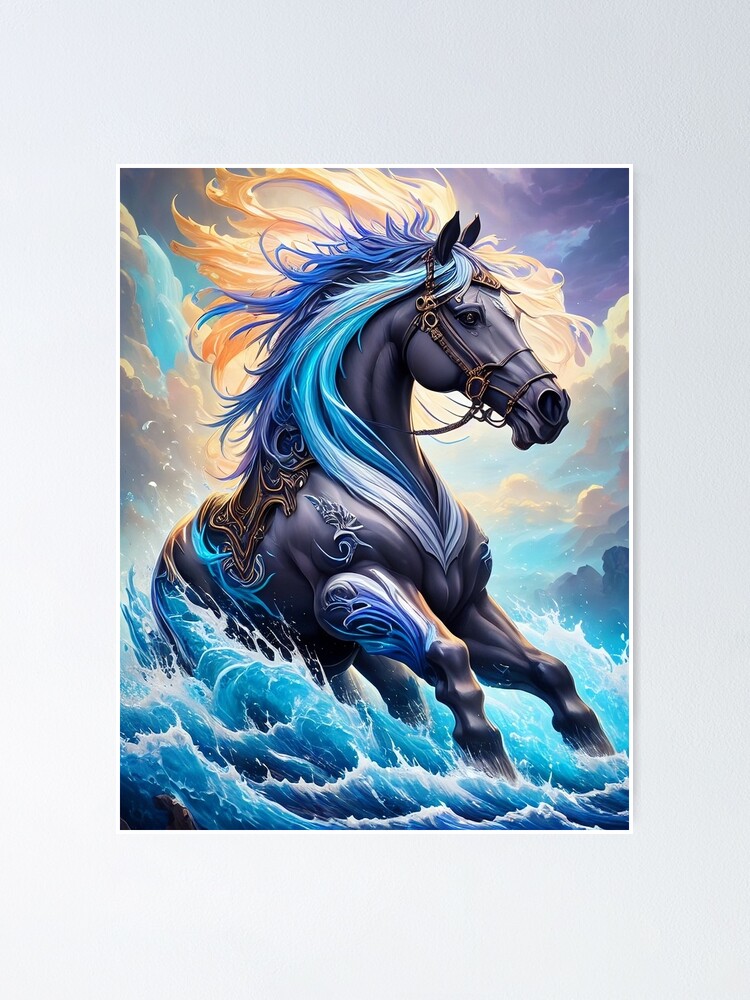This captivating five-by-seven art piece features a stunning gray stallion charging through a splashing expanse of blue water, set against a pale gray wall with a thin white border framing it. The horse, highlighted in various shades of gray and purple, is adorned with an ornate golden bridle that wraps around its face and continues down its back as part of a decorative saddle. Its mane is a vivid blend of colors: dark blue streaks fly upwards, mingling with purplish blue strands, and vibrant neon green or turquoise hair cascades down its neck, catching the sunlight and lending a golden sheen. The scene is dynamic, with water splashing around the horse's legs, captured in intricate detail with smaller whitecaps crowning the splashes. To the right, larger white water splashes complement the horse's powerful movement. In the background, misty hills and a sky with dramatic hues of light blue, purple, and gray create a stunning backdrop, further accentuated by streaks of white and orange behind and above the horse. This masterpiece conveys a sense of energy and grandeur, with the horse depicted as a majestic creature in a moment of dynamic action.